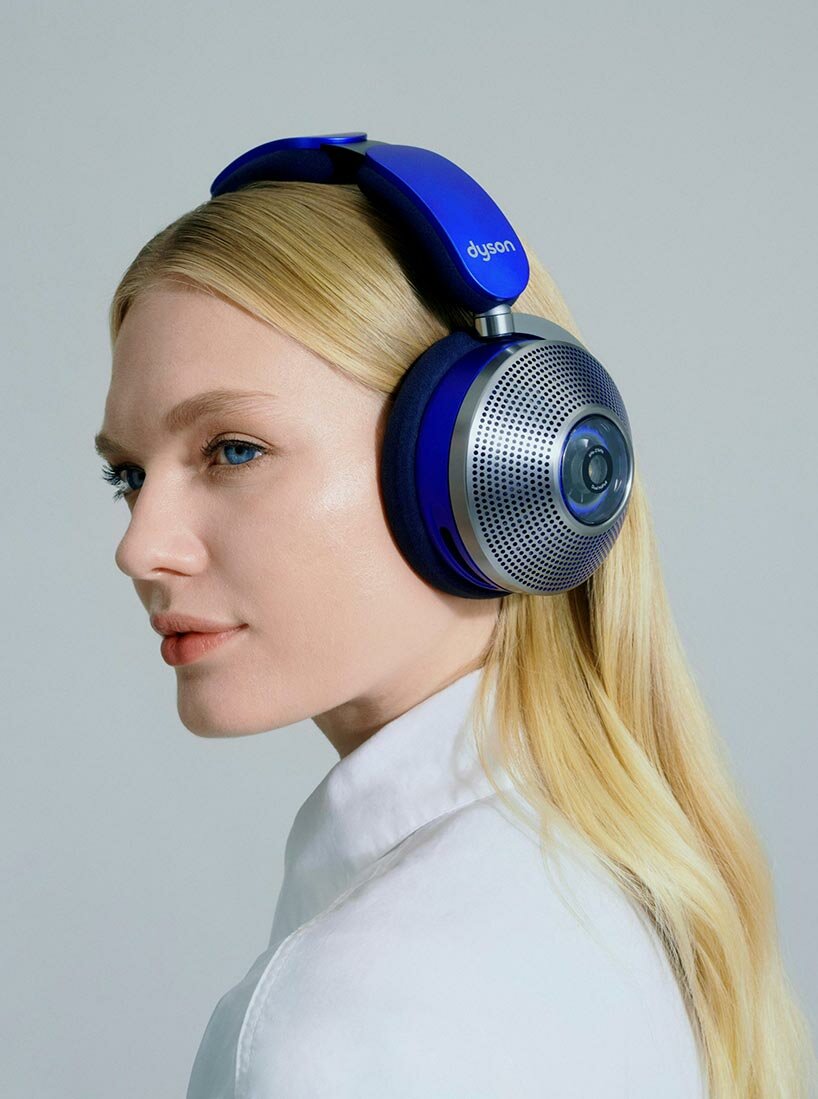This detailed photograph, likely from an advertisement, features a young, blonde woman with blue eyes and fair skin, set against a gradient greenish-gray background. She is dressed in a white shirt and is the focal point of the image. The most striking element is the pair of Dyson headphones she wears. These headphones are a deep, vibrant blue transitioning to brushed silver on the earpieces. The silver sections are punctured with evenly spaced tiny holes and potentially feature a small window, giving a glimpse of the internal speaker. The headband of the headset prominently displays the Dyson brand in silver letters. The overall composition highlights the sophisticated design of the headphones, almost as blue as the woman's captivating eyes.